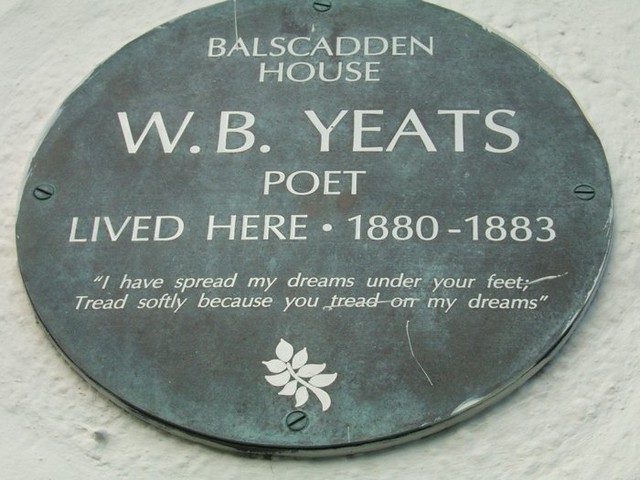The image features a single, centrally positioned round plaque set against a sandy-colored, possibly stone or concrete, background. The metallic, green plaque is affixed to the surface with matching rivets or screws. Detailed white text on the plaque reads: "Balscotton House. W.B. Yeats, poet, lived here 1880 to 1883. 'I have spread my dreams under your feet; tread softly because you tread on my dreams.'" Additionally, there is an image of a branch with leaves etched into the plaque in the same color as the text. The scene appears to be an outdoor historical site, captured in broad daylight, portraying a realistic setting that emphasizes the text and the historical relevance of the location.